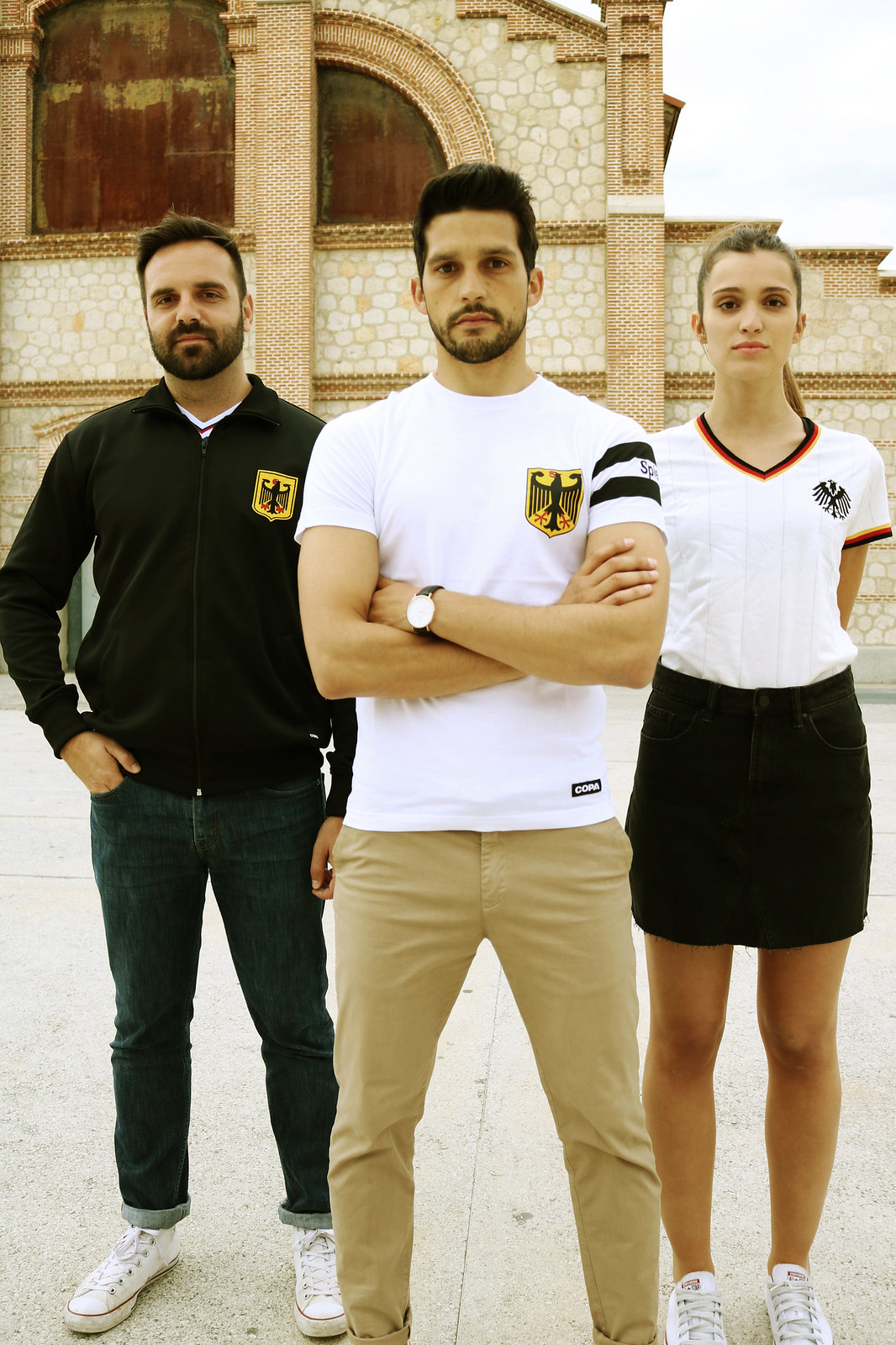In this outdoor image, three individuals stand confidently side-by-side in front of a rustic stone brick building with aged, golden-tinted windows. The sky is mostly cloudy, with a small hint of blue visible in the upper right-hand corner. The central figure is a man wearing a white short-sleeved shirt with a black and white stripe on one arm, paired with tan pants. To his right stands a girl in a black skirt and white V-neck polo shirt, her hair neatly pulled back, and she is wearing white tennis shoes. To the left is another man dressed in a long-sleeved black shirt, blue jeans, and white tennis shoes, notable for his beard, similar to the central figure. They all appear to be modeling soccer merchandise, likely for a German team, given the red, yellow, and black colors themed with their attire. Their poised demeanor and careful styling suggest they are posing for a promotional image, possibly for a magazine or an online website.